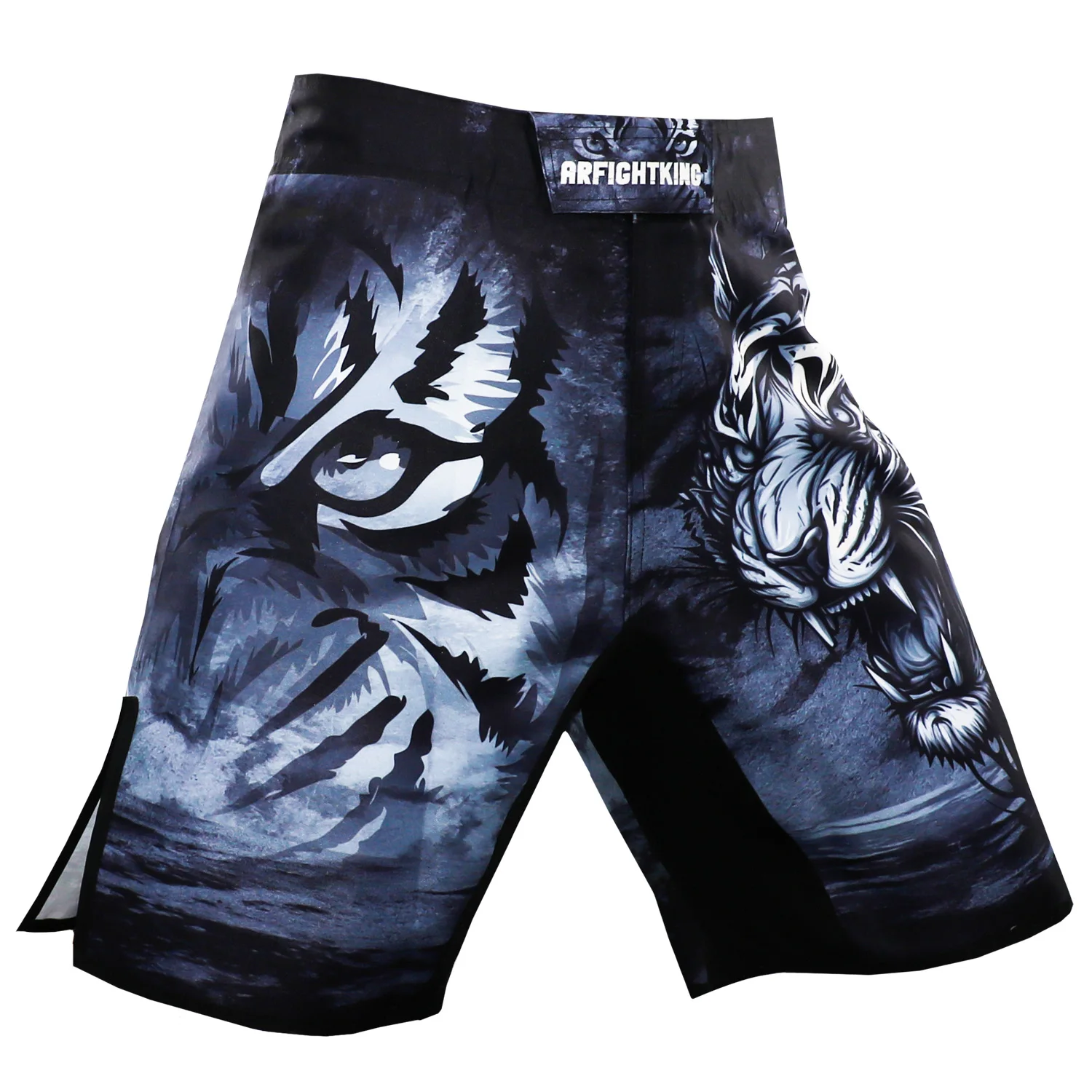This image showcases a pair of athletic shorts, likely designed for boxing or UFC, featuring visually striking graphics. The shorts predominantly exhibit a bluish-black color scheme with black seams and small slits on both outer leg areas. The waistband is black, with white text in the center that reads "AR Fight King." On the left leg, there's a detailed depiction of a tiger's face, with only one eye clearly visible. Contrastingly, the right leg displays a full tiger's head, mouth open in a growl, showcasing sharp fangs and fierce expression. The tiger, rendered in blue, black, and white, adds a bold and dynamic aesthetic to the shorts.